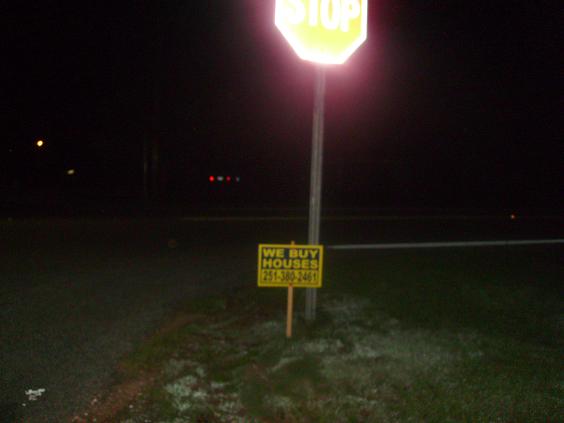In this blurry, out-of-focus nighttime photograph, the main subject at the center is a standard red stop sign with white lettering mounted on a metal pole that extends to the top of the image. Just below the stop sign is a yellow advertisement sign with a black box and yellow writing that reads, "We Buy Houses," followed by a phone number, which is partly legible as 2513802461. The backdrop is a dark night sky. The setting appears to be an open field or a front yard, characterized by areas of dying grass interspersed with dirt, gray cement, and some rocks. In the upper left corner, there is a hint of reflecting light, possibly from distant brake lights of a car. The street depicted seems to split off, forming a T-intersection, suggesting potential left and right turns.